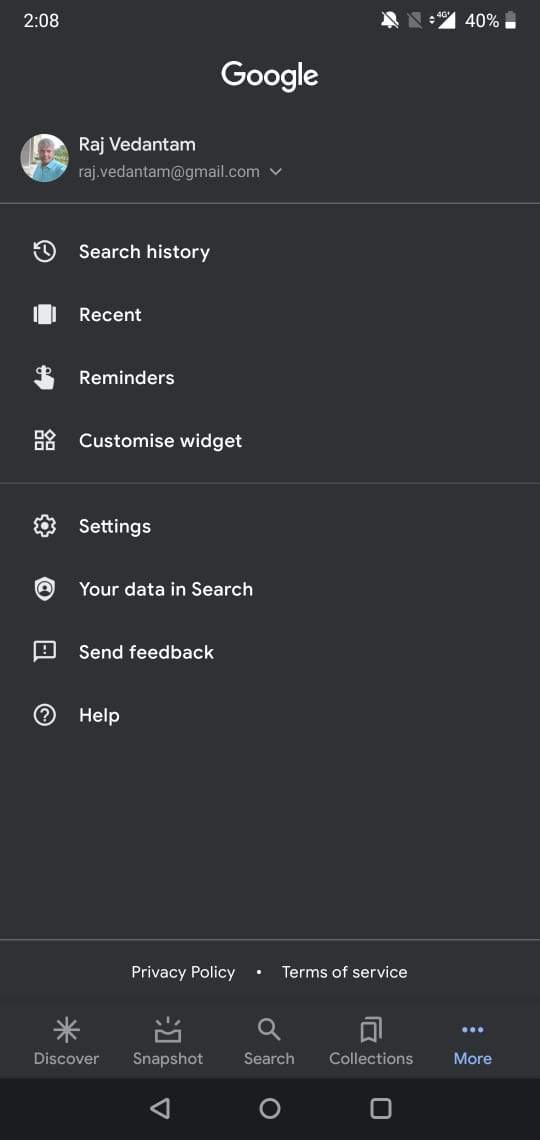This is a detailed screenshot from a smartphone with a sleek black and white user interface. The background is entirely black, providing a clear contrast to the white text and icons. 

At the top of the screen, the number "208" is prominently displayed. To the right of this number, a crossed-out bell icon indicates that notifications are turned off. The status bar also displays the coverage icon and the battery level, which is currently at 40%.

Centered at the top is the word "Google," followed by the email address "Raj Vedantam, R-A-J dot V-E-D-A-N-T-A-M at gmail.com" in clear text. To the left of the email address is a small, circular photo of a man smiling directly at the camera.

Below this section, a list of options is presented in white text:
- Search History
- Recent
- Reminders
- Customize Widget
- Settings
- Your Data in Search
- Send Feedback
- Help
- Privacy Policy
- Terms of Service
- Discover
- Snapshot
- Search
- Collections
- More

At the very bottom of the screenshot is a black banner featuring three icons: a white left-pointing arrow, a circle, and a square.

The dimensions of the image are taller than they are wide. The screenshot is notably devoid of any animals, birds, plants, flowers, trees, or automobiles.